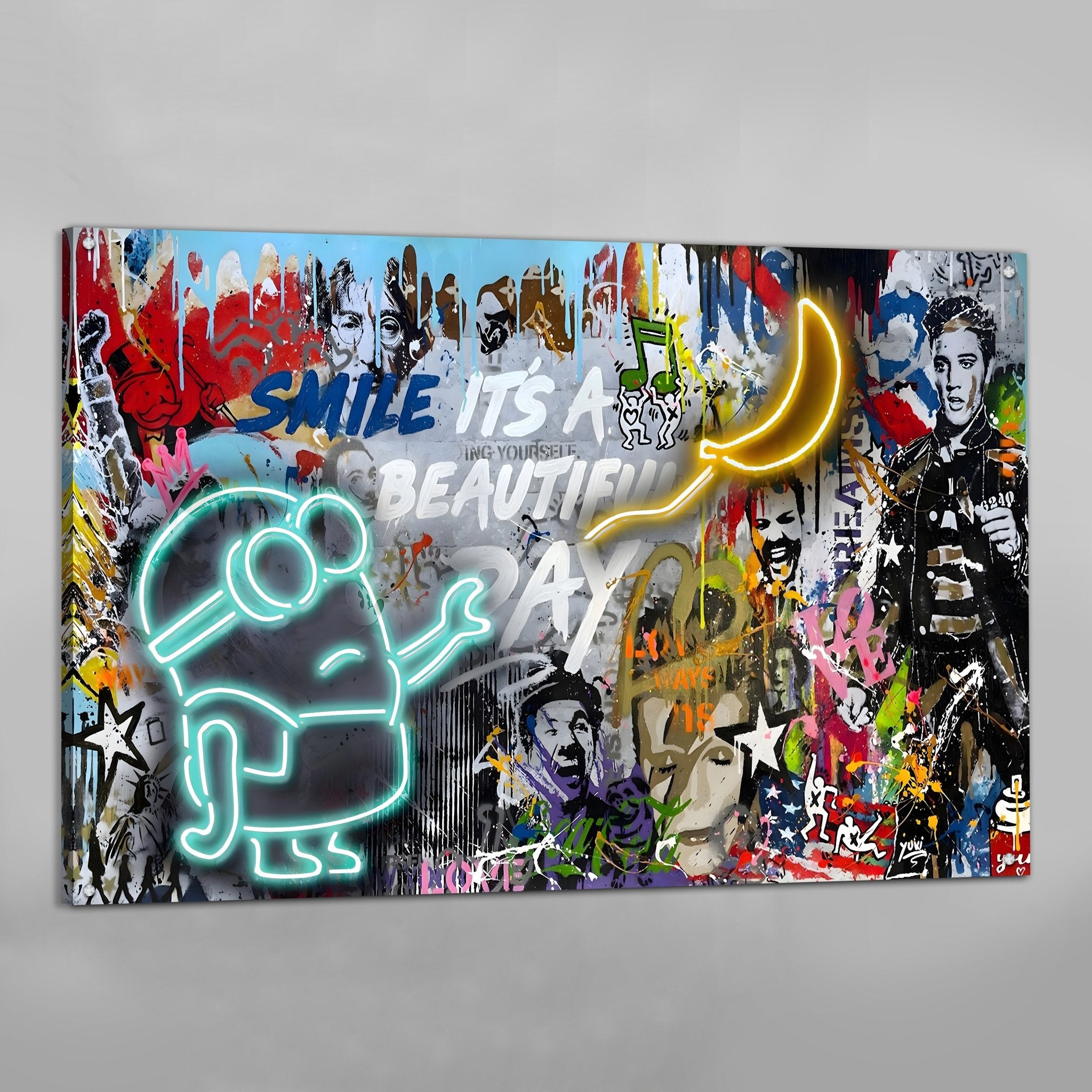The vibrant, unframed painting on a medium light gray canvas is bursting with eclectic imagery and vibrant colors, reminiscent of a graffiti mural. Centered in the artwork, the words "Smile, it's a beautiful day" are prominently featured, with "smile" written in striking blue and the rest in white. A neon-style minion, outlined in teal and facing right, appears to be reaching out toward a yellow balloon that resembles a banana. This minion adds a playful, whimsical touch to the piece.

The background is layered with a chaotic yet captivating array of faces and symbols, all splattered with an energetic mix of pink, blue, black, and red paint. Notable figures include the Mona Lisa, Charlie Chaplin, a glam pop singer, Queen Victoria, and the Monopoly man. Elvis Presley takes up much of the right side of the painting, while above him, a man with a black mustache is discernible. Intermixed with these characters are additional elements like a gold heart, a star, an American flag, and a spray paint can at the bottom, adding to the painting’s vibrant complexity.

The overall composition is a dense collage of familiar cultural icons and abstract forms, creating a rich tapestry that invites viewers to discover new details with every glance.